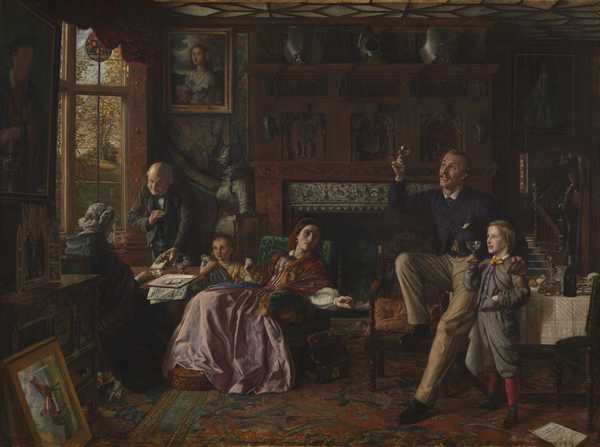This painting, dating back to the 18th century, depicts a detailed indoor scene involving multiple figures, likely representing a family gathering. The foreground is dominated by a man in a black suit coat and white shirt, standing by a wooden window with brown borders. This man appears to be serving a woman seated at a wooden table to his right. The woman, with gray hair and clad in a black shawl, sits alongside an old man who leans forward near the window.

Adjacent to this pair, another grouping captures attention: a woman in a long pink dress, which flows past her ankles, sits in a green chair. A young girl stands close by. Both are near a large fireplace with a wooden mantel adorned with horizontal marble accents.

In the right section of the painting, an adult man wearing a blue sweater and light pants, sporting a mustache, sits next to a young boy dressed in a gray suit with red socks and black shoes. This boy, holding a glass goblet in his right hand, stands in front of a wooden table draped with a white tablecloth. Both the man and the boy are depicted with a raised right hand, as though toasting. Stairs ascend in the background towards the right corner of the room, completing this rich tableau of historical familial interaction.